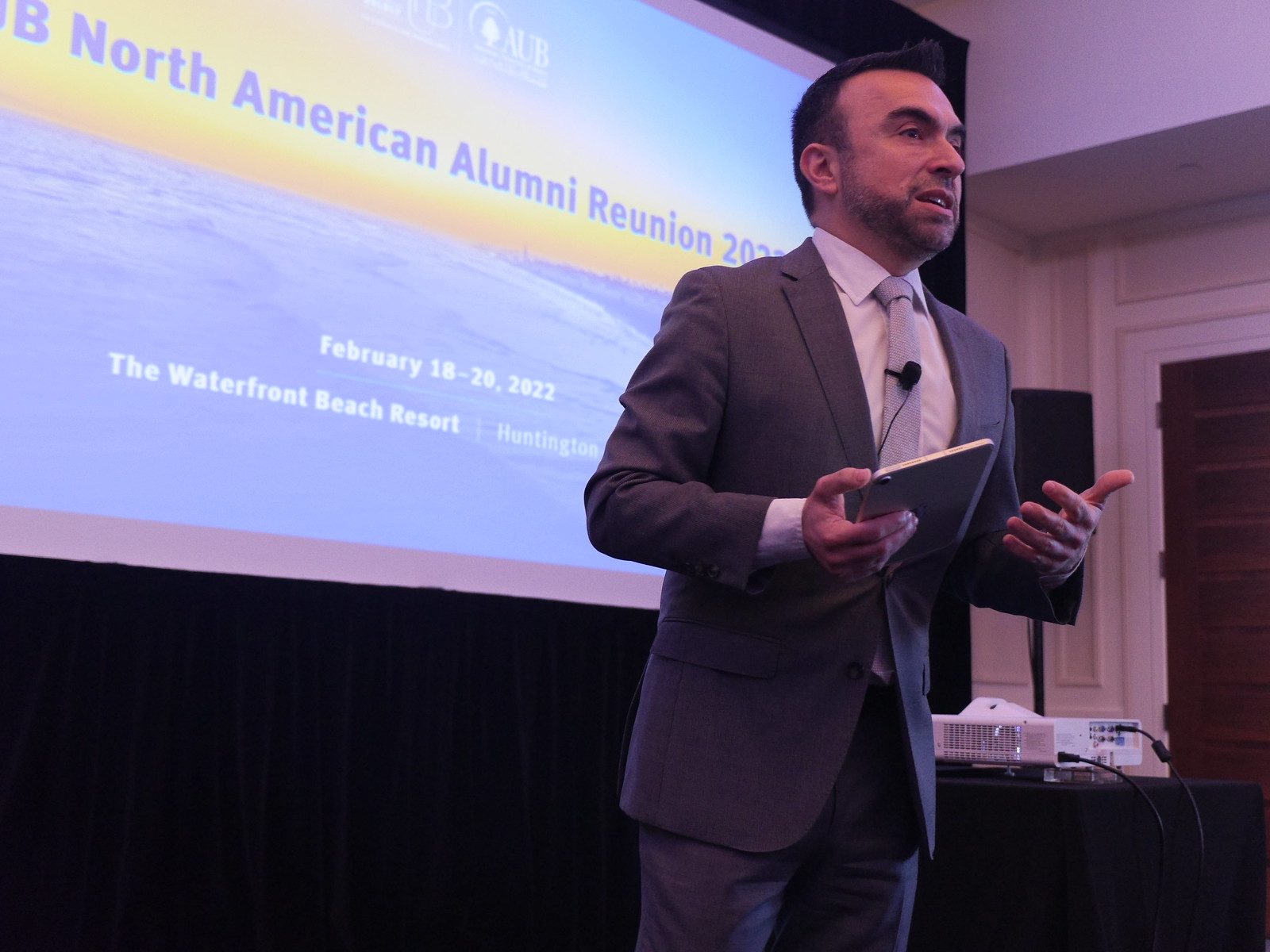In the image, a well-dressed man stands slightly off-center, wearing a gray suit with a white undershirt and a light blue tie, which is adorned with a black clip-on microphone. He has brown hair and a brown beard, and he holds a gray tablet in his right hand. The setting appears to be an event space, perhaps a boardroom or classroom, where he is giving a speech. The text on the projector screen behind him reads, "North American Alumni Reunion February 18th to 20th, 2022 at the Waterfront Beach Resort, Huntington." To the right of the man, a white projector rests on a table, with a speaker mounted above it, adjacent to a brown door and a white wall. The projector screen displays a mix of blue, yellow, and white colors, aligning with the text. The man is likely discussing plans for the upcoming reunion event.